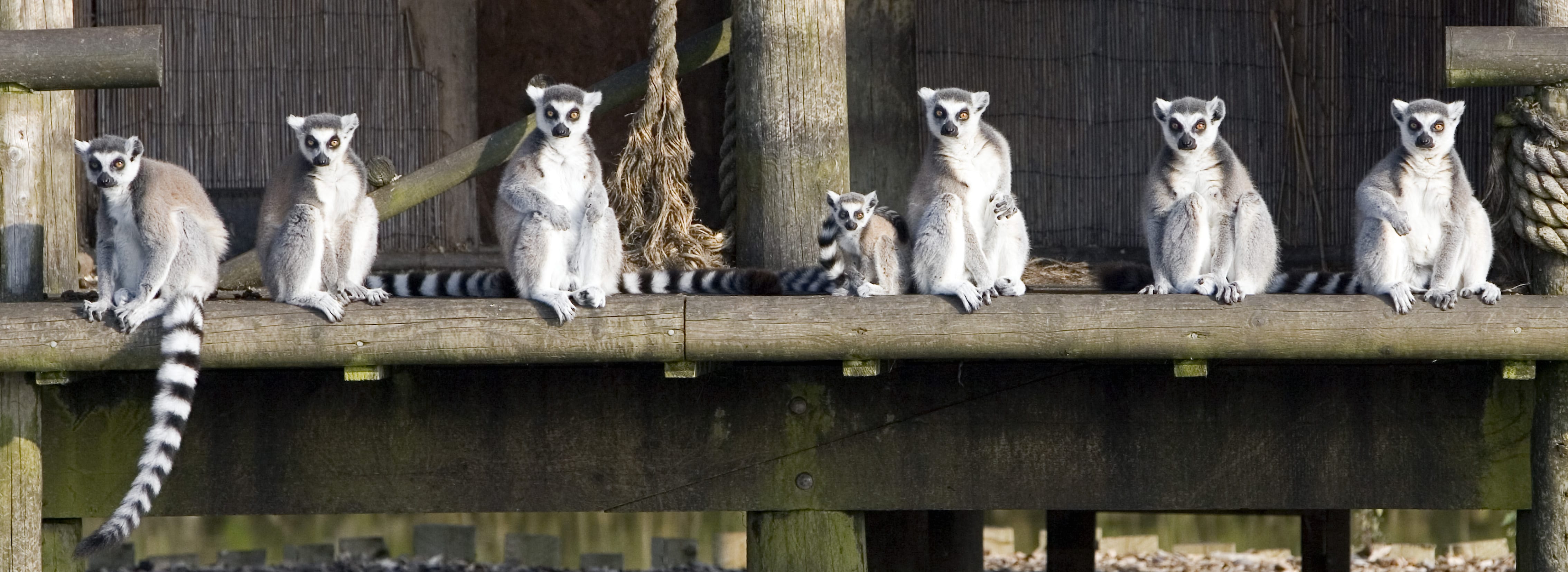In this captivating image, seven ring-tailed lemurs, including one baby, are perched on a rustic wooden structure. Their striking black and white ringed tails drape gracefully around them. Each lemur is covered in mostly white fur with distinctive dark markings: black around their yellow eyes, on their noses, and along their tails. They all sit attentively and stare directly into the camera, their gazes intense and almost inquisitive.

The lemurs are positioned on a log that stretches across the image from left to right. One lemur’s tail dangles off the front, while another tail rests across the baby lemur’s back. The log is part of a larger, somewhat primitive structure, featuring a tall wooden pillar at the center and a frayed rope hanging down. The backdrop hints at a partial view of a building, possibly a barn or a museum exhibit, with moss growing at the base, adding to the natural atmosphere. The photograph catches a moment where these curious creatures seem to engage directly with the viewer, creating a profound connection.